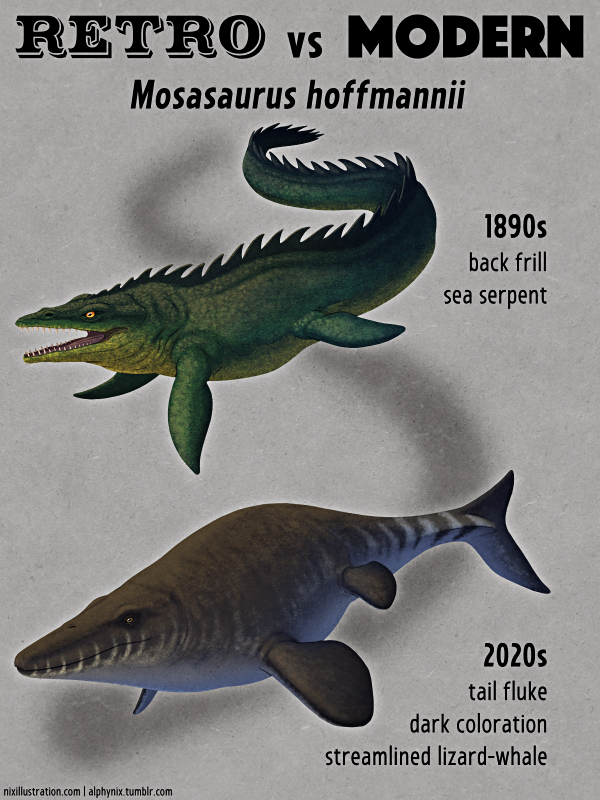This vertical rectangular poster with a grayish background features bold black text at the upper left that reads "RETRO VS. MODERN." Just below this header, the scientific name "Mosasaurus Hoffmannii" is prominently displayed. The poster visually compares two versions of this prehistoric creature. The upper image showcases an 1890s depiction labeled "Back Frill Sea Serpent," portraying a dark green creature resembling an alligator with pointed scales along its back, a spiked tail, and a menacing open mouth filled with sharp teeth, complemented by striking yellow eyes. In contrast, the lower image features a modern interpretation from the 2020s called "Tail Fluke." This version is described as a streamlined lizard whale, predominantly dark gray with a light gray underside and subtle stripes. It has a closed mouth and dark eyes with yellow accents, exhibiting a less menacing but more realistic representation. The modern creature has two sets of fins and a tail, emphasizing a sleek, aquatic design. The poster employs mostly neutral colors with standout green and yellow details to highlight the evolutionary contrast between the two depictions.